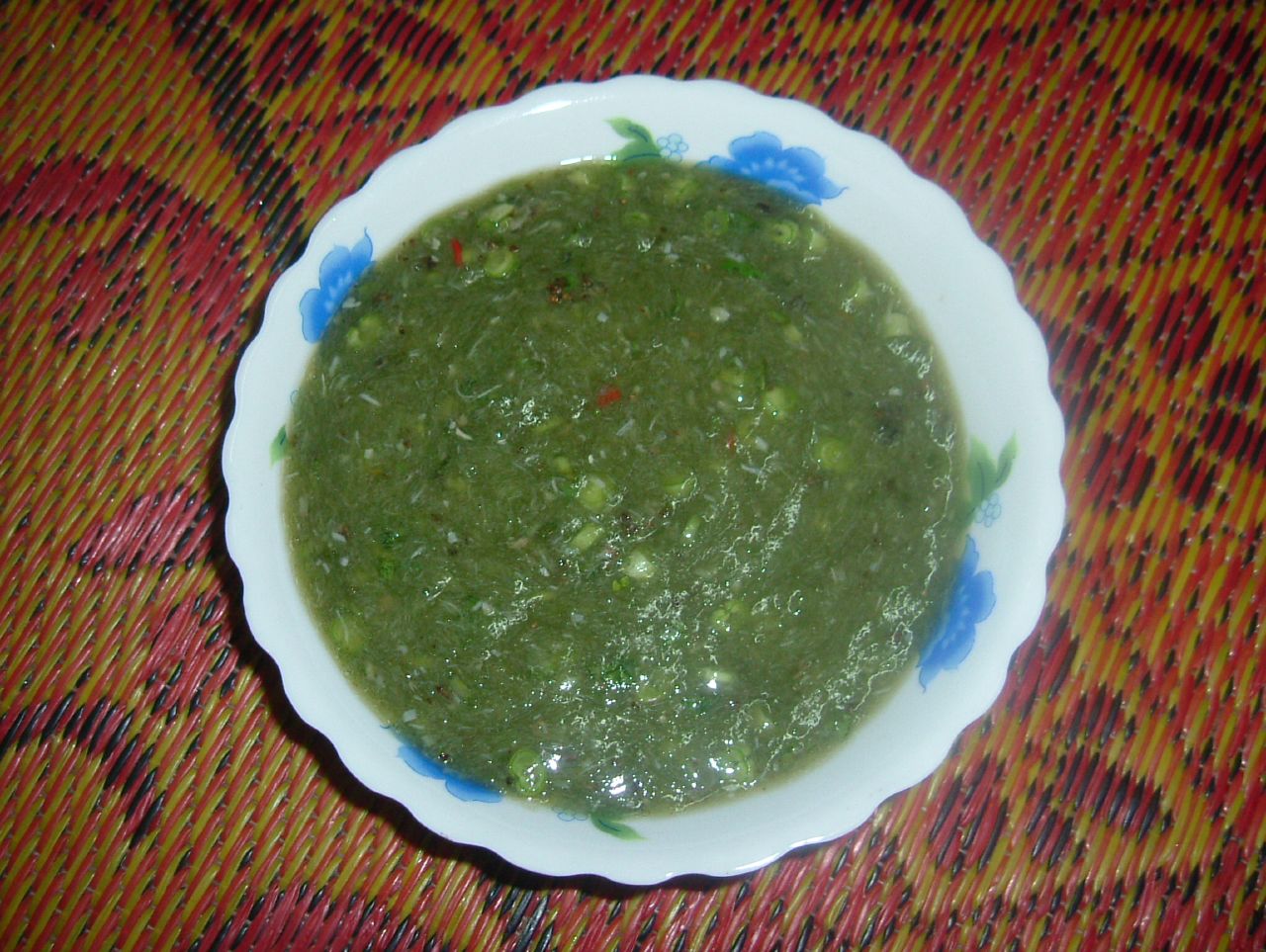The image features a top-down view of a white plate with wavy edges, adorned with blue floral motifs. The plate is resting on a brown bamboo surface with red flower patterns and intricate line designs. Inside the plate is a vividly green soup or sauce, possibly spinach-based, containing various ingredients. There are visible red pieces that could be tomatoes, green onions, and tiny white pieces which might be rice or other small ingredients. The plate, detailed with its blue flowers, complements the multi-colored tabletop design featuring a red, yellow, and black stitched floral pattern, adding to the rich visual tapestry of the scene.